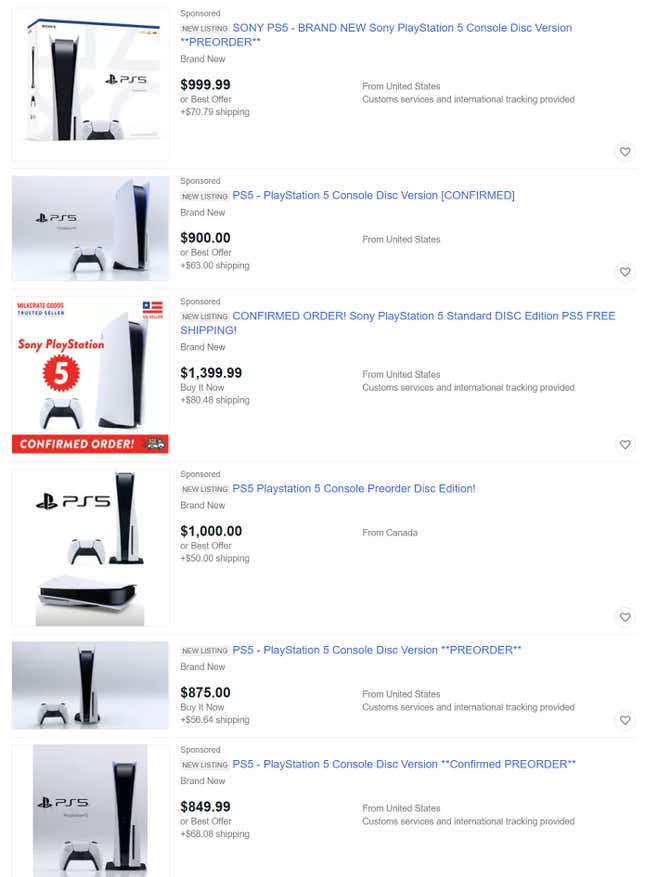A crisp webpage screenshot showcasing various product listings against a clean white background. Each entry features a square product image on the left, followed by a light gray rectangle with dark gray, uppercase text reading "NEW LISTING." To the right of this rectangle, a blue title with detailed product information is displayed.

The highlighted listing at the top depicts a box featuring a black and white image of a video game console. On its right, above the "NEW LISTING" box, dark gray text indicates "SPONSORED." The adjacent blue text reads "Sony PS5 - Brand New Sony PlayStation 5 Console Disk Version," followed by asterisks and the uppercase word **PREORDER**. Below this, light gray text states "brand new," followed by bold black numerals showing the price "$999.99." Beneath the price, light gray text indicates "or best offer" and "+ $70.79 shipping." Further details include "from United States," and "custom services and international tracking provided," with a circular light gray heart icon in the bottom right corner.

The subsequent listing features a different image, displaying the console itself outside of the box. It also includes the "SPONSORED" and "NEW LISTING" text. The classified title is "PS5 - PlayStation 5 Console Disk Version [CONFIRMED]." It mentions "brand new," with a price tag of "$900.00," an option for "or best offer," and shipping costs of "+ $63.00." The final note at the bottom right reads "from United States." The listings continue in a similar, structured fashion throughout the page.